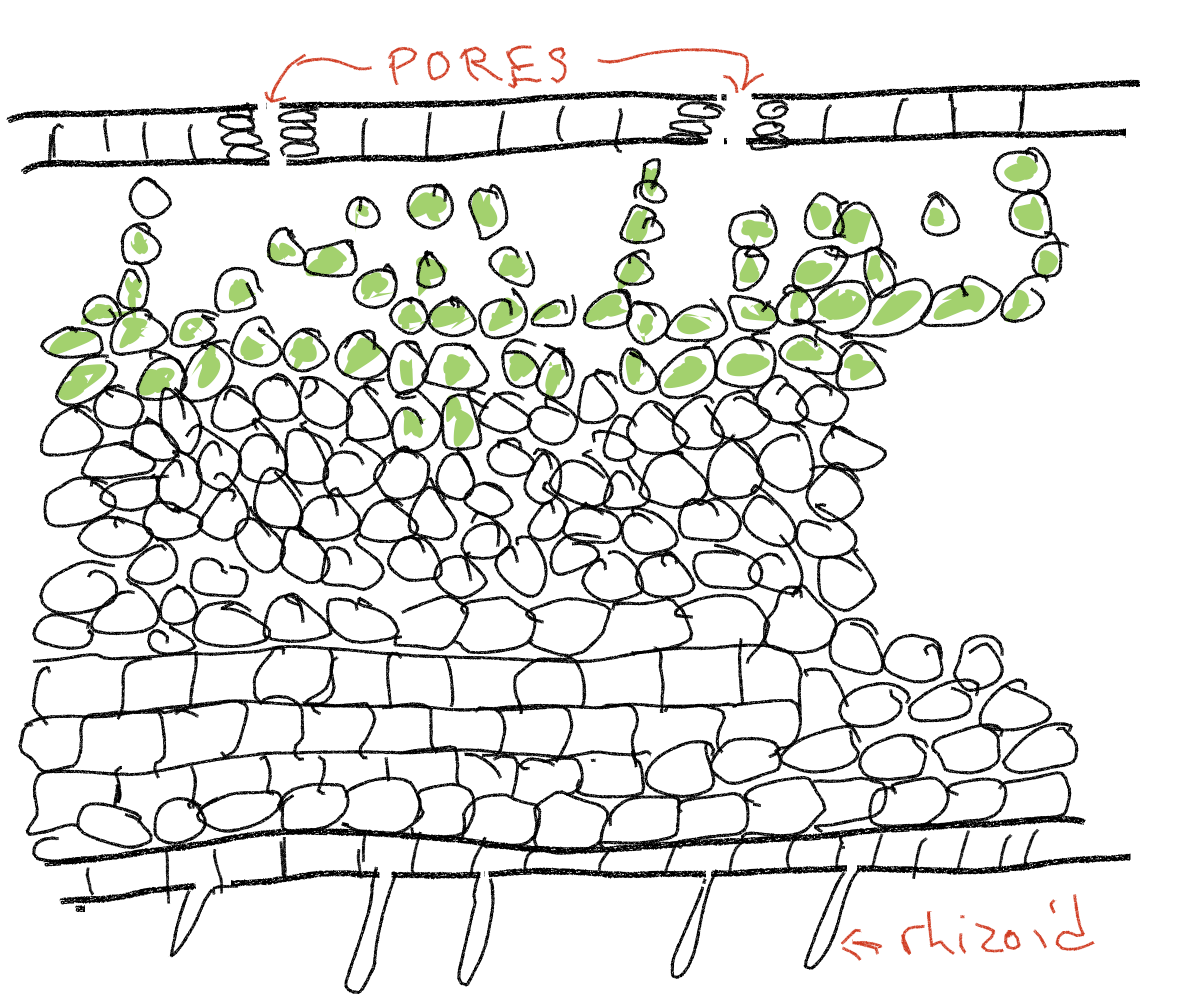This image is an amateurish sketch, likely by a student for a biology class, portraying the structure of what appears to be plant cell walls. The top of the drawing is labeled "pores" in red letters, pointing to illustrated openings. Just beneath these pores, there are layers of circular plant cells, some colored in green ink, situated underneath what might be a layer of skin or similar structure. Further down, additional circles remain uncolored, drawn solely with black ink, representing different layers of cells. At the bottom, another section of the drawing is labeled "rhizoid" in red letters with an arrow pointing towards structures that extend from the wall, which are likely the roots of the cells. This detailed, hand-drawn scientific illustration combines various labels and annotations, aiming to explain the anatomy of plant cells and their formations.